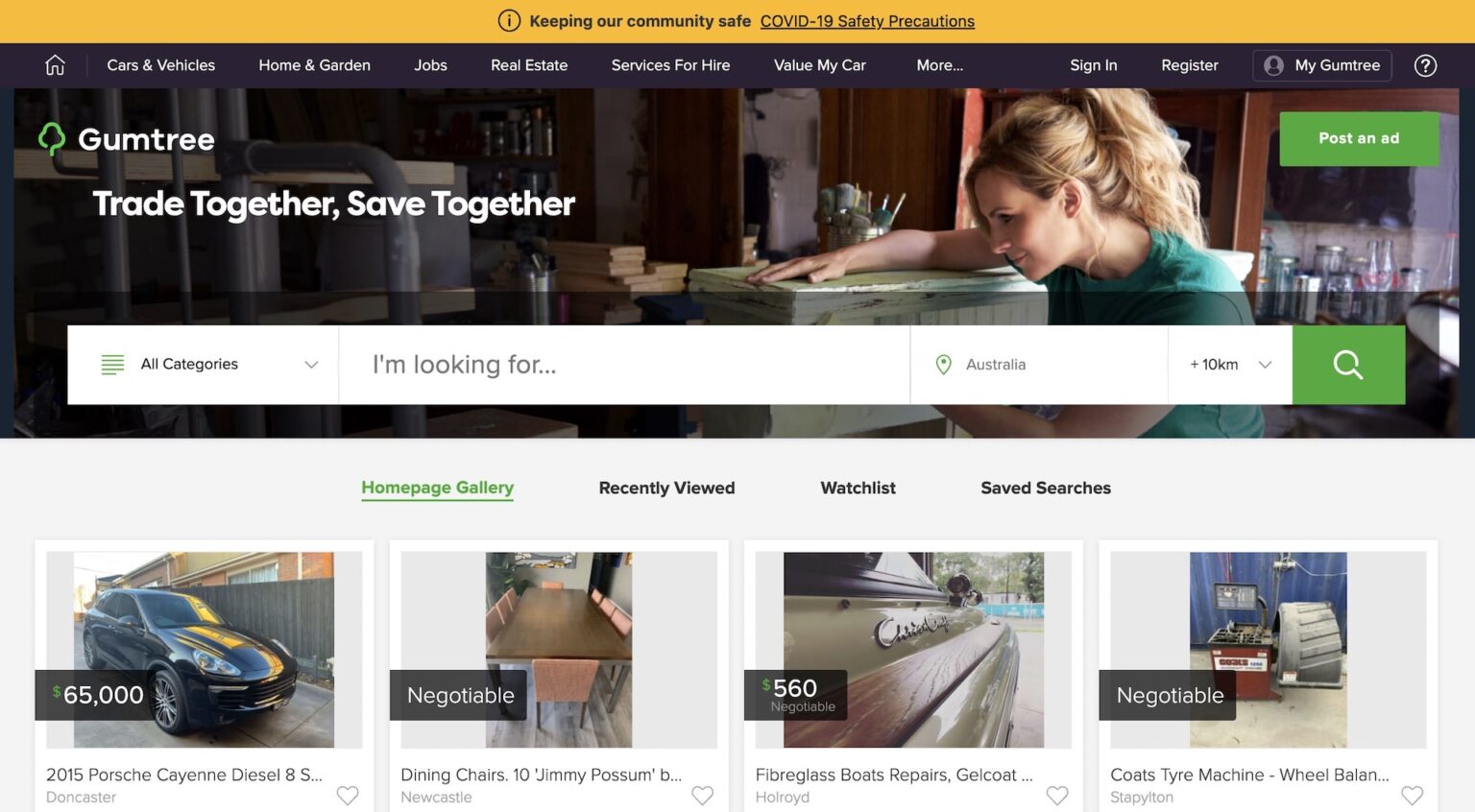A detailed caption for the image could be:

"The image captures the screen of a web page from a platform called Gumtree. At the top of the page, there's a green icon featuring a tree next to the site's name, conveying the theme 'trade together, save together.' A yellow rectangle with rounded edges sits at the top, bearing a tiny lowercase 'i' inside a circle, and it highlights an important message: 'Keeping our community safe: COVID-19 safety precautions.' Below this header, the navigation bar includes various categories like 'Cars & Vehicles,' 'Home & Garden,' 'Jobs,' 'Real Estate,' 'Services for Hire,' 'Value My Car,' and a 'More...' option indicated by an ellipsis.

To the right, account-related options such as 'Sign in,' 'Register,' and 'My Gumtree' are visible. The main section of the page features an image of a woman who appears to be closing a box while intently examining it, suggesting some form of engagement with a product or item. Around her, green buttons labeled 'Post an Ad' are positioned for user interaction.

A search bar lies below, with placeholders reading 'All Categories,' 'I'm looking for…,' 'Australia,' and 'within 10 km,' encouraging users to refine their searches. At the bottom, four rectangular boxes list items with price tags marked as 'Negotiable,' indicating the flexibility in pricing."